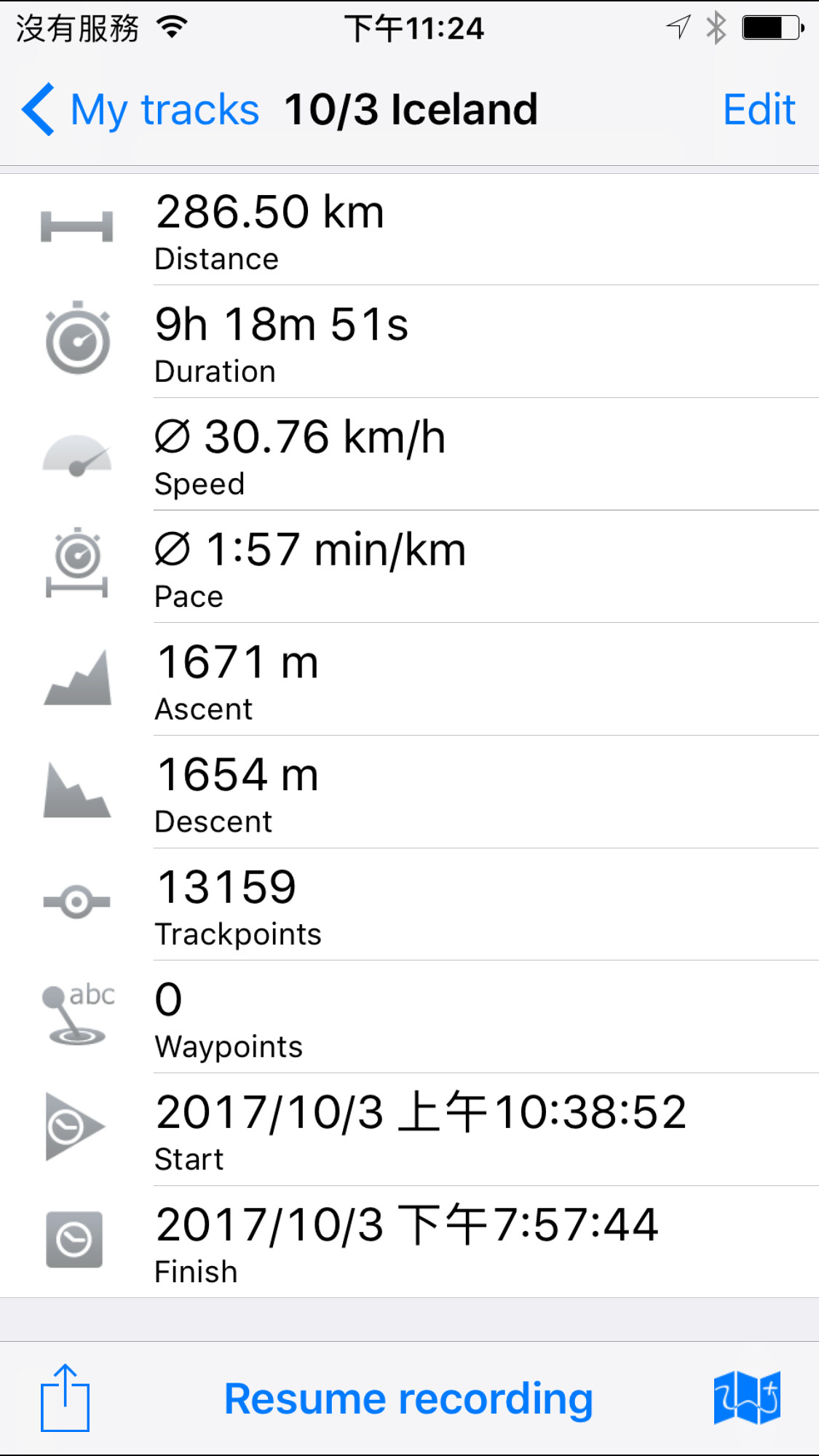This is a detailed screenshot from an iPhone, primarily in Japanese. The top left corner displays Japanese characters and Wi-Fi signal bars, with the time "11:24" in the middle. To the right, there's an arrow icon and a battery indicator showing about 70% charge. Below that, there's a blue arrow next to "My Tracks 10/3 Iceland," with an "Edit" option in blue text to the right. Continuing down, there's a left column of icons followed by corresponding text. The icons include an "H" with "286.50 kilometers distance," a clock showing "9 hours 18 minutes 51 seconds duration," a speedometer with "30.76 kilometers per hour speed," an alarm clock with an "H" depicting "157 minutes per kilometer pace," a mountain with "1671 meters ascent," a descending mountain with "1654 meters descent," a circle with "1350/159 track points," a joystick with "ABC" indicating zero waypoints, an arrow with a clock and numbers labeled "start," and a square with a clock and numbers labeled "finish." At the bottom, there's a blue share logo with "resume recording," and to the right, a map icon. The screen background is white with black text, with the listed metrics possibly pertaining to a race or tracking activity.